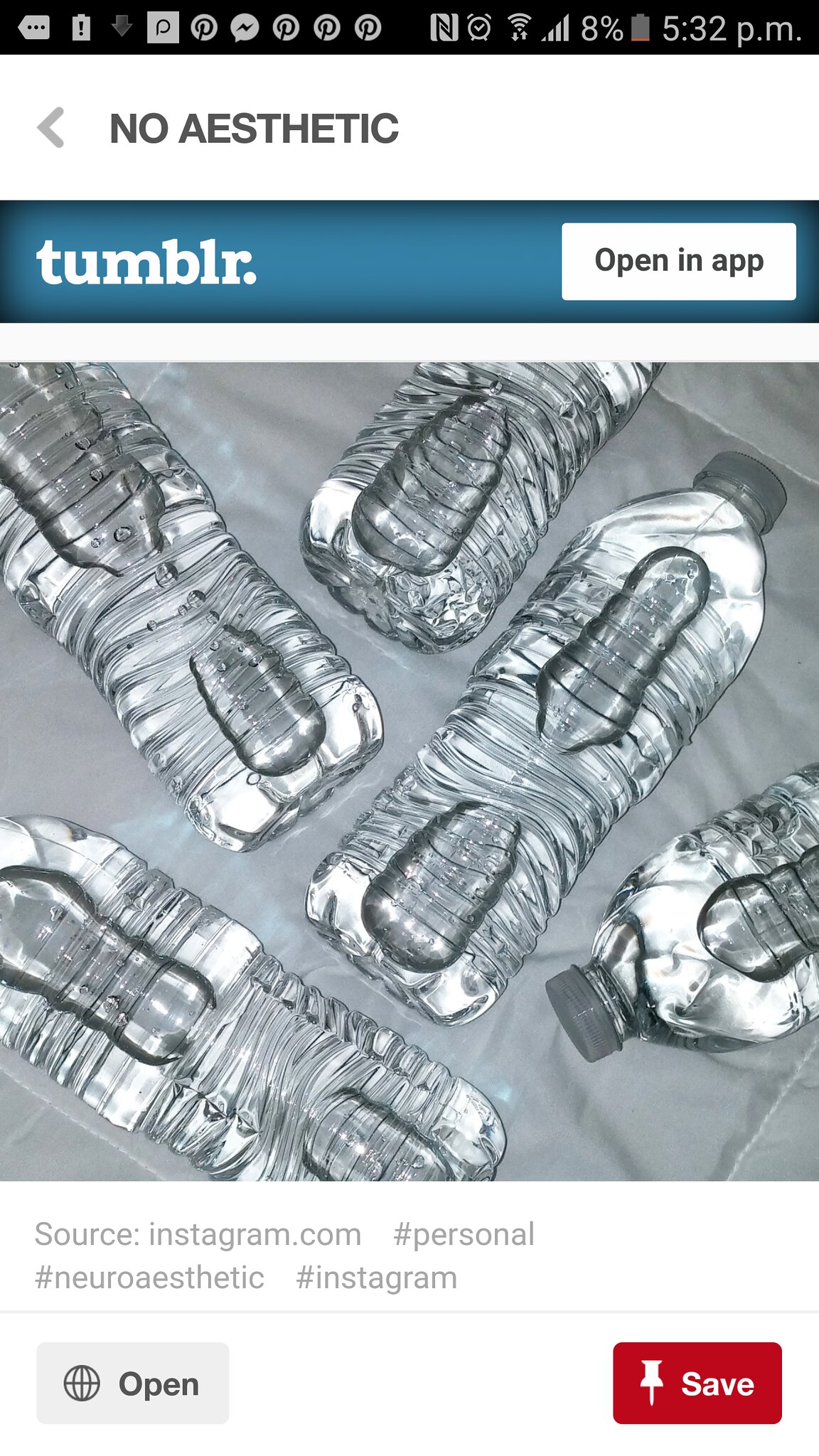The image is a detailed color screenshot taken from a smartphone, as indicated by the black bar at the top showing familiar icons. On the top right, the time is 5:32 PM, next to a mostly grey battery icon with a small red bar and an 8% remaining battery indication, signaling low power. Other icons, all white, include a signal strength indicator, a Wi-Fi symbol, an alarm clock, and a near-field communication (NFC) icon. Various notifications appear on the left, such as a Pinterest icon and a message icon with a lightning bolt.

The main screen captures a Tumblr post sourced from Instagram, featuring an image of several clear plastic water bottles with grey screw-on lids, arranged randomly and without labels. Each bottle contains water and, due to their horizontal position, air bubbles are visible within them. These bottles appear to be lying in a clear tray filled with water. 

At the top left of the screenshot, the words "No Aesthetic" are visible with a left-pointing arrow, acting as a back button. Further below, there's a blue rectangular area with the Tumblr logo ("tumblr.") and a white button with black text that says "Open in app." At the bottom right, a red rounded rectangle with a drawing pin icon is labeled "Save." The text below the image includes tags like hashtag personal, hashtag neuro aesthetic, and hashtag Instagram, suggesting an Instagram origin for the photo.